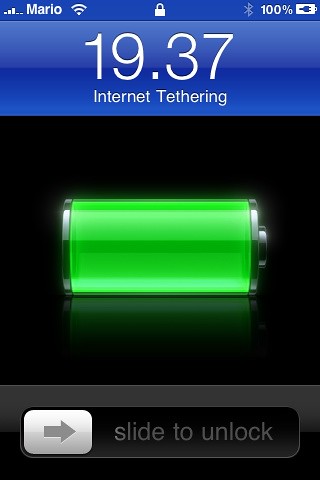This image displays a screenshot from an iOS device, likely an iPhone, captured at its lock screen. At the top, the name "Mario" appears in white text, accompanied by signal bars, a Wi-Fi icon, a lock symbol, and a 100% battery indicator all on a blue background. Below this, in lighter blue, the time is shown as "19:37", with "Internet Tethering" written beneath it in white text. Central to the image is a black box housing a bright green battery icon with silver edges, appearing reflective and glowing against the black background. At the bottom, a gray banner reads "slide to unlock" in small, gray text beside a right-pointing arrow within a white square. The composition suggests the vibrant lock screen of an iOS device.